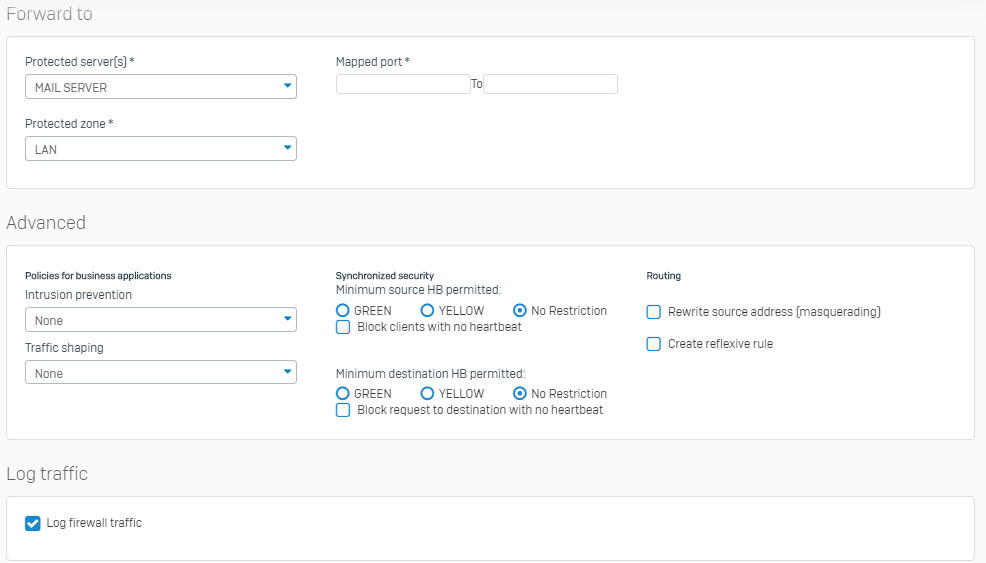The image depicts a detailed panel for email setup options, divided into three distinct sections, each highlighted with light gray headers and white panels bordered by thin pixel lines.

1. **Forward To**:
   - Below the light gray header "Forward To", there are options for configuring protected servers. 
   - "Mail Server" is displayed in uppercase with a drop-down menu next to it, marked by an asterisk indicating a required field. 
   - Following this, "Protected Zone" is another drop-down menu labeled with an asterisk, where "LAN" is currently selected.
   - To the right of these options is the "Mapped Port" field, also marked with an asterisk, accompanied by input fields for specifying the port numbers.

2. **Advanced**:
   - Under the "Advanced" section, policies for business applications can be configured.
   - There are drop-down options titled "Choosing Prevention" and "Non-Traffic Shipping", both set to "none".
   - To the right, a column labeled "Synchronized Security" displays configurable options, including:
     - "Minimum Security to HP Permitted" with the selections: "Green", "Yellow", and "No Restriction". The latter is currently selected.
     - "Block Clients with No Heartbeat" option, which is unchecked.
   - Similarly, "Minimum Destination HP Permitted" is presented with the same selectable options and current selection.
   - Further to the right, under the "Routing" section, there are two unchecked options:
     - "Rewrite Source Address (Masquerading)"
     - "Create Reflexive Rule"

3. **Log Traffic**:
   - The bottom section labeled "Log Traffic" features a blue check mark beside the text "Log Firewall Traffic," indicating that this option is enabled.

All these elements are displayed on a clean, white background.

This detailed structuring allows for comprehensive email setup and security management, with clearly defined options and selectable fields for user customization.